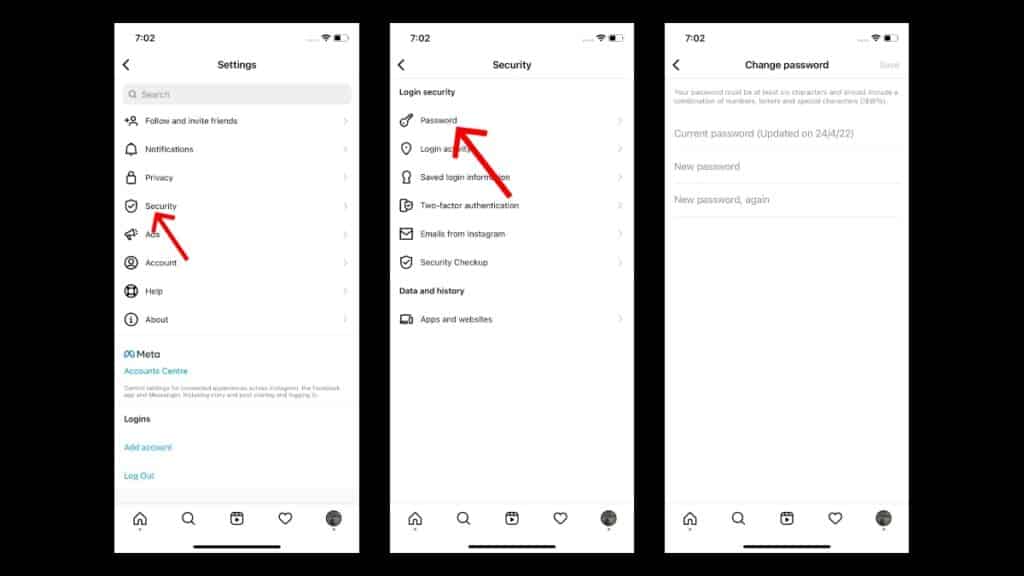**Caption:**
A step-by-step tutorial on updating your password, presented in a series of three screenshots against a black background. 

1. The first screenshot displays the phone's settings menu with multiple options. A prominent red arrow points to the "Security" option, signified by a black-font label and an icon resembling a badge with a checkmark.

2. The second screenshot shows the security settings screen. Various security choices are presented, and a red arrow highlights the "Password" option, which is identified by a key icon.

3. The final screenshot details the password update interface. It provides information about the last password update and offers instructions on how to create a new password. 

The sequence of red arrows guides users clearly through each step, ensuring an easy navigation from accessing settings to updating the password.